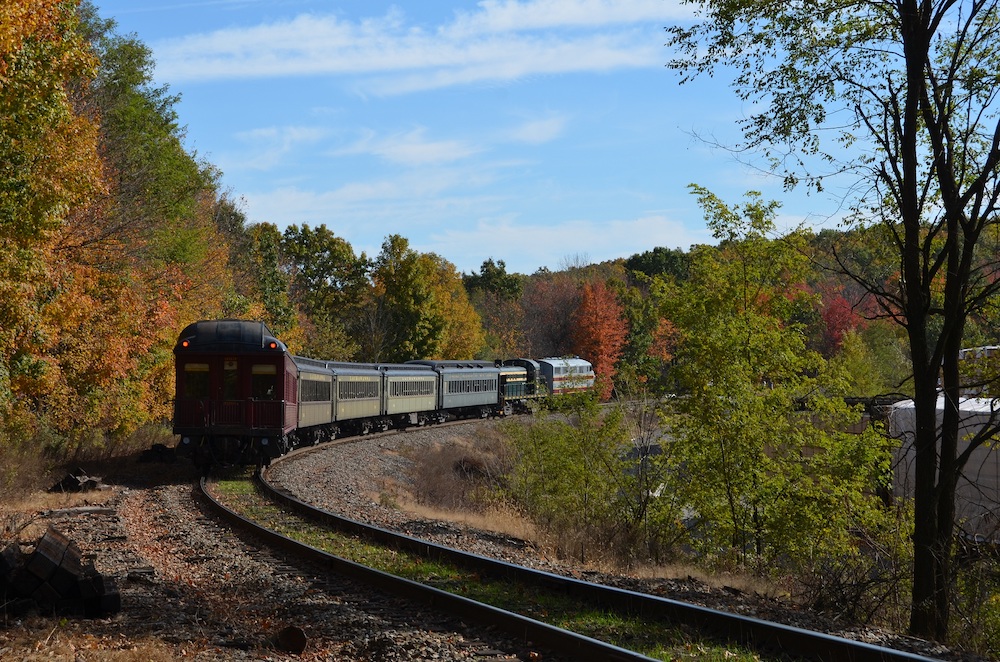This vibrant autumn photograph captures a picturesque scene of a train journeying through a hillside adorned with vivid foliage. At the top of the image, a pale blue sky kissed by wispy, cirrus clouds contrasts beautifully with the array of red, orange, yellow, and green trees that blanket the hills below. In the middle of the frame, a red locomotive pulls a series of train cars—gray, blue, green, yellow, and pale silver—along winding tracks. The train, rounding a curve, appears to be heading towards the camera, creating a dynamic focal point. The tracks, starting from the bottom right corner, curve gracefully through the landscape, accompanied by green and mostly leafless trees on either side. In the backdrop, a hint of a white building or vehicle peeks through the dense, colorful foliage. This rich and detailed scene impeccably captures the essence of autumn's beauty, with the train adding an element of movement and life to the serene landscape.